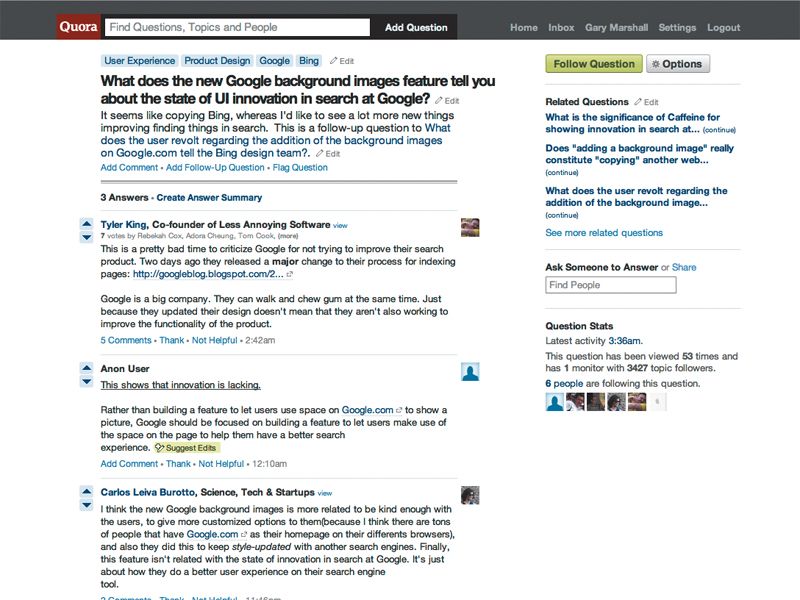This image displays a webpage resembling a search or explorer interface, bearing the branding "Cura" at the top left within a red rectangle, with "Cura" written in white text. Below this, there's a search bar prompting users to "Find questions, topics, and people," alongside an "Add Question" button.

On the top right, navigation options are visible, including "Home," "Index," "Gary Marshall," "Settings," and "Layout." Central to the page, several topics are highlighted in blue: "User Experience," "Product Design," "Google," and "Bing." 

Directly below, an article headline reads: "What does the new Google background images feature tell you about the state of UI innovation in search at Google?" The subsequent text suggests that this feature appears to be mirroring Bing's approach, expressing a desire for more innovation in search enhancements.

This article is positioned as a follow-up to a previous question about user reactions to Google’s addition of background images and its implications for Bing's design team. Below the article, three answers are presented with an option to "Create Answer Summary." One of the contributors is identified as Tyler King, co-founder of "Lemp's Annoying Software." 

On the sidebar, additional related questions are listed, providing further context and continuity to the ongoing discussion threads.